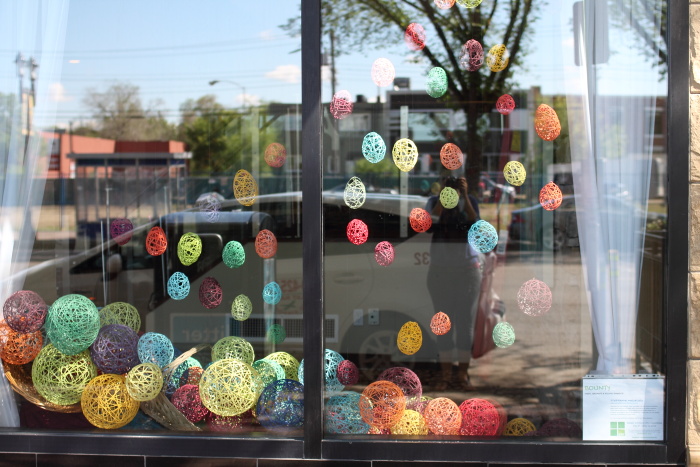This color photograph showcases a large, double-pane retail display window adorned with an intricately arranged assortment of vibrant, hanging ornaments. These egg-shaped decorations, made from colorful plastic or a meshed material, dangle from the ceiling in hues ranging from orange, red, yellow, green, blue, purple, and peach. An estimated fifty ornaments hang above a collection of transparent, spherical ornaments at the bottom of the display. The scene suggests an Easter celebration theme.

The window’s reflective surface prominently captures the external environment: the photographer, a woman standing in front of a small white car, is visibly reflected alongside another building, a tree, and the blue daytime sky with a scattering of clouds.